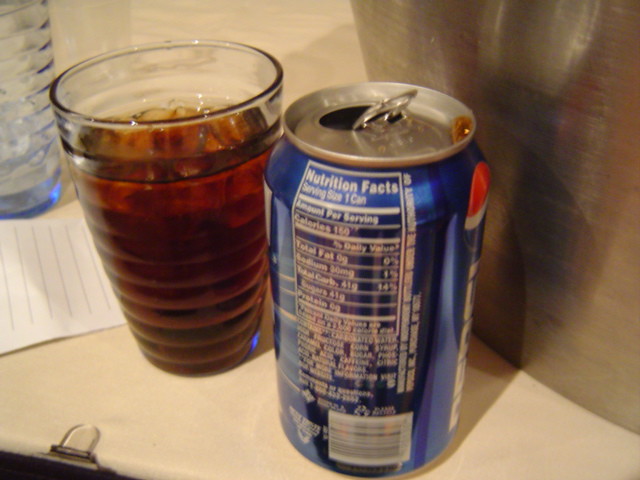In this captured image, a can of Pepsi, oriented to display the Nutrition Facts, is positioned prominently on a thin, beige Formica table in the corner of a room. Adjacent to the can, slightly in the background, stands an elegant glass adorned with spiral patterns, filled with ice-cold Pepsi. Also visible in the background are an empty, lined piece of paper, which may be a receipt, and a water bottle. The scene is partitioned, hinting at a corner table setup.